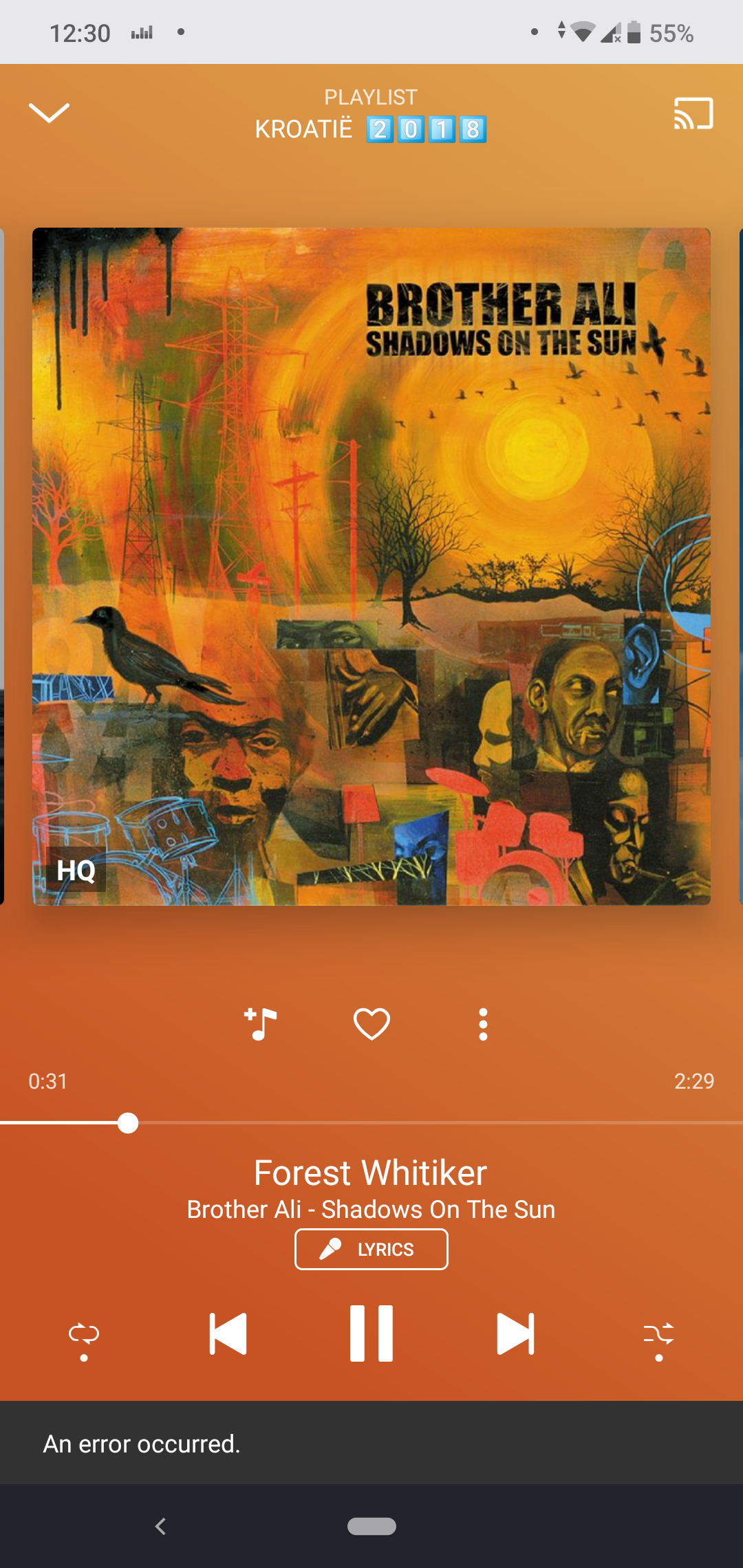The image appears to be a screenshot taken from a cell phone, with a gray bar at the top displaying the time as 12:30 in the left corner and a battery life of 55% on the right side, along with a vertical black bar indicating signal strength. Below this bar, the background color transitions to burnt orange. In the center, "Playlist" is displayed in white text, followed by "K-R-O-A-T-I-E" underneath, and four small blue squares beside it.

The main part of the image features what resembles the cover art for an album or a theme for music, depicting a variety of elements: a small black crow positioned with the sun behind it, several men's faces at the bottom, a randomly placed blue ear, some long red lines, black branch-like trees, a pathway, and birds flying away from the sun. In black text, it reads "Brother Ali, Shadows of the Sun."

The bottom section of the image shows a music player interface indicating that a song is currently being played, with a progress bar at 0:51 out of a total duration of 2:29. Below this, the song title "Forest Whitaker" by Brother Ali from the album "Shadows of the Sun" is displayed.